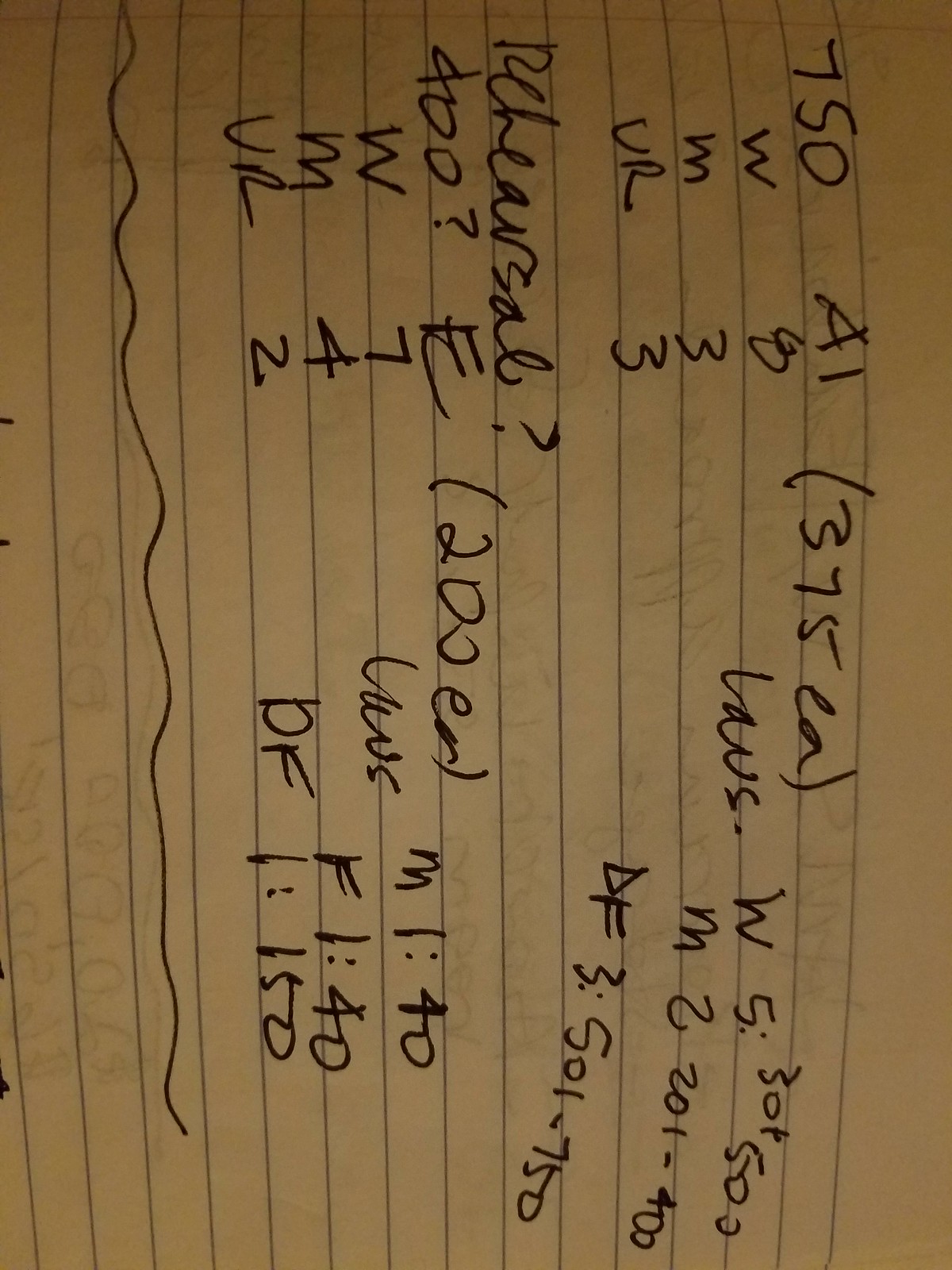This image depicts a piece of white notebook paper with blue horizontal lines. The text is written in black ink and appears sideways, requiring the viewer to rotate their head or device to read it properly. The writing is partially legible and covers less than half of the page. 

Prominently, the text includes fragmented codes and numbers such as "750 AI," which is followed by "375 EA" in commas. Beneath that, it reads "W8. M3 UR3 LAVS." On the opposite side, there's "W5 30T5." Other visible text includes "M2 201-400" and "DF3 501-750." Below these, there's a phrase "rehearsal?" followed by "400?" and "E 200 ER" in parentheses.

Additional notes feature sequences like "W7 M4 UR2 LAVS M1; 40," "F1; 40," and "DF1; 150," all separated by semi-colons. A squiggly line is drawn underneath all the written content. Slight transparency allows for the faint visibility of text from the back side of the paper.